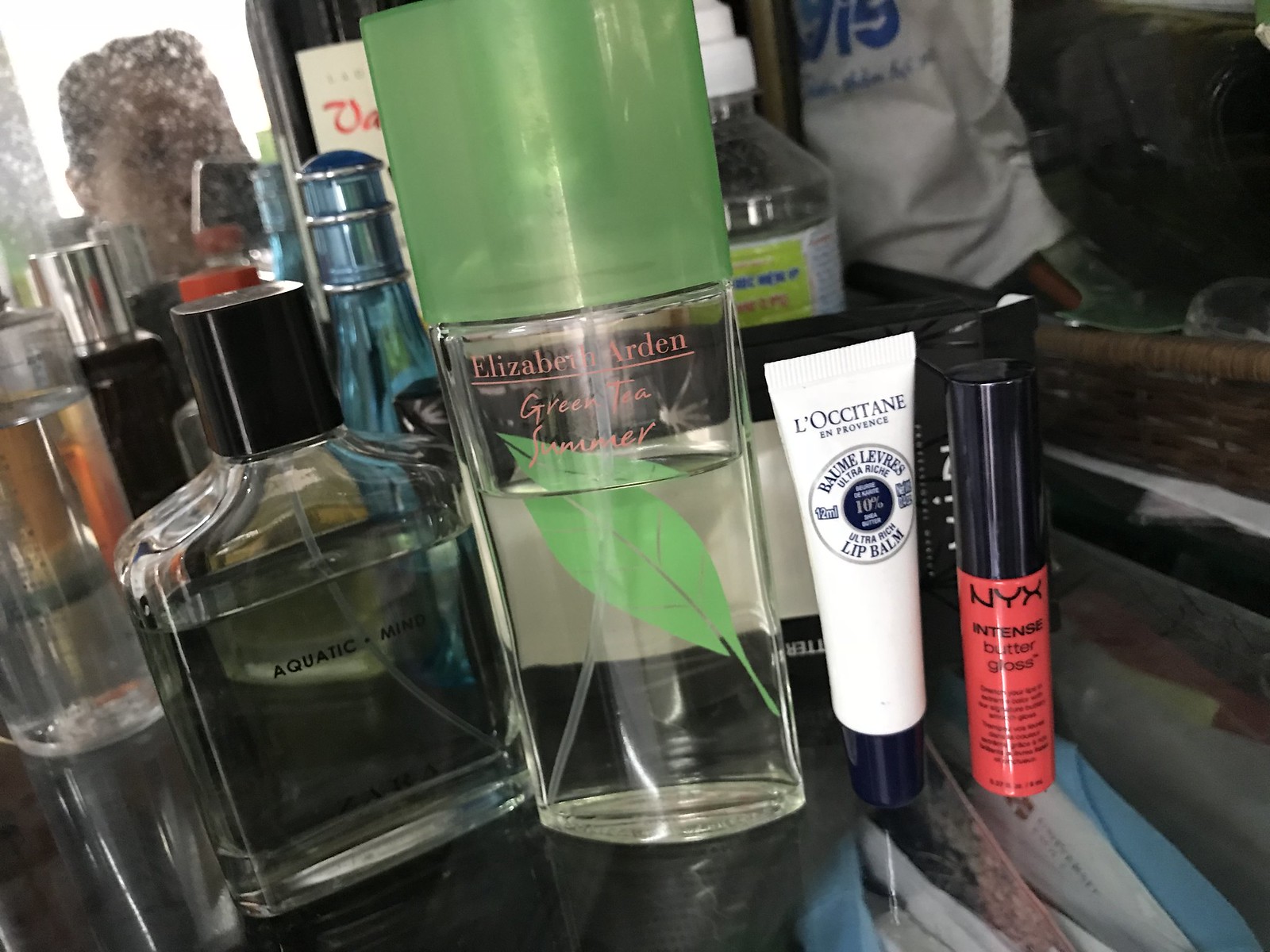The image depicts a cluttered tabletop, possibly in a bathroom or a bedroom. Spread across the surface are various personal care items including a lip balm labeled "butter gloss" with an "aquatic mint" flavor, an aftershave, and a glass of water. To the right, there's a mirror which adds to the ambiguity about whether the location is a nightstand or a dresser. The mirrored reflection hints at another bag placed nearby. To the left, another mirror or possibly a window, reflecting a man who appears to be looking at his phone, though the view is unclear due to the dirt and spots on the glass. Below the tabletop, newspapers are visible underneath a glass surface, adding to the overall disarray and mystery of the setting.